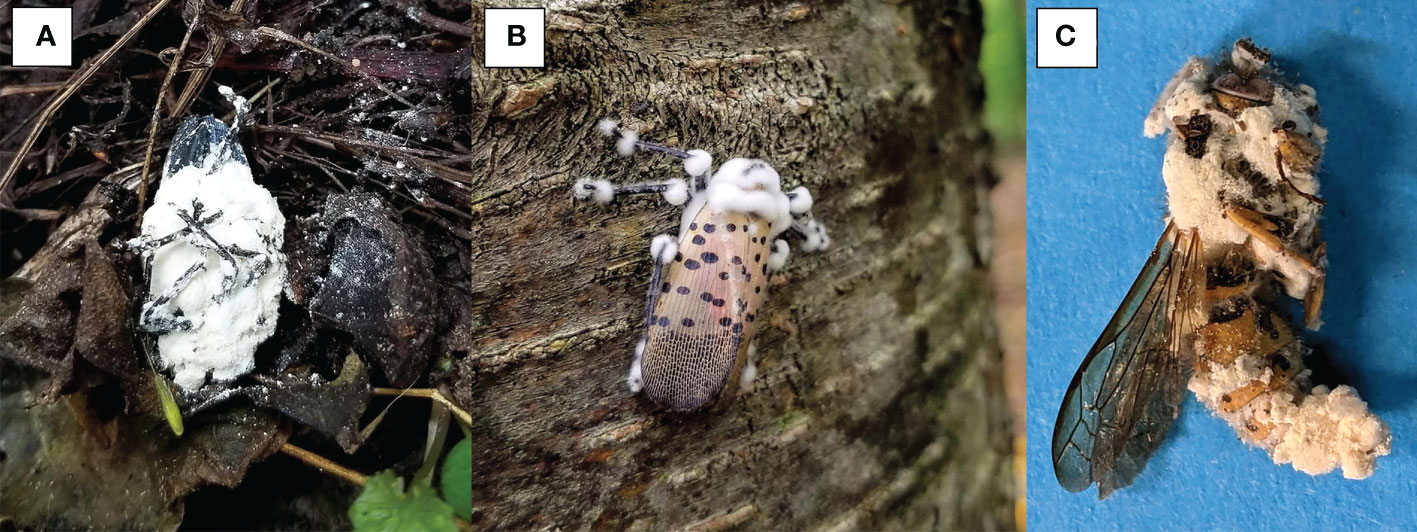The image is a collage of three photographs, each depicting different stages of an insect's life cycle, labeled A, B, and C within a white square with a black border. 

In the image labeled A on the left, a black insect, possibly a larva or early-stage pupa, is positioned in what appears to be a dry plant. This insect is covered in a white, mold-like substance. 

The middle photograph, labeled B, shows a dotted beetle or insect with furry legs climbing on a tree trunk.

The final image, labeled C, displays an insect that resembles a bee or wasp with a light yellow body, crusted with what appears to be remnants of wings. It is lying on a light blue foam-like surface, suggesting it may be dead or decomposing.